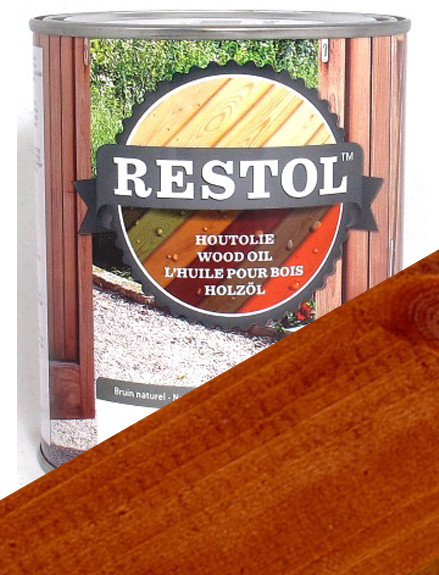The image depicts a color photograph of a large, round can with a silver lid, set against a white wall. The can prominently features the label "RESTOL," spelled in all caps with a trademark symbol. Above the RESTOL branding, the label shows untreated planks of light brown wood, while below it, stained wood in various strong, vibrant colors is displayed. The text "WOOD OIL" is visible on the label, repeated in multiple languages. In the foreground, a richly stained, grainy wooden board extends across the bottom right corner of the image, showcasing the effect of the wood oil product.